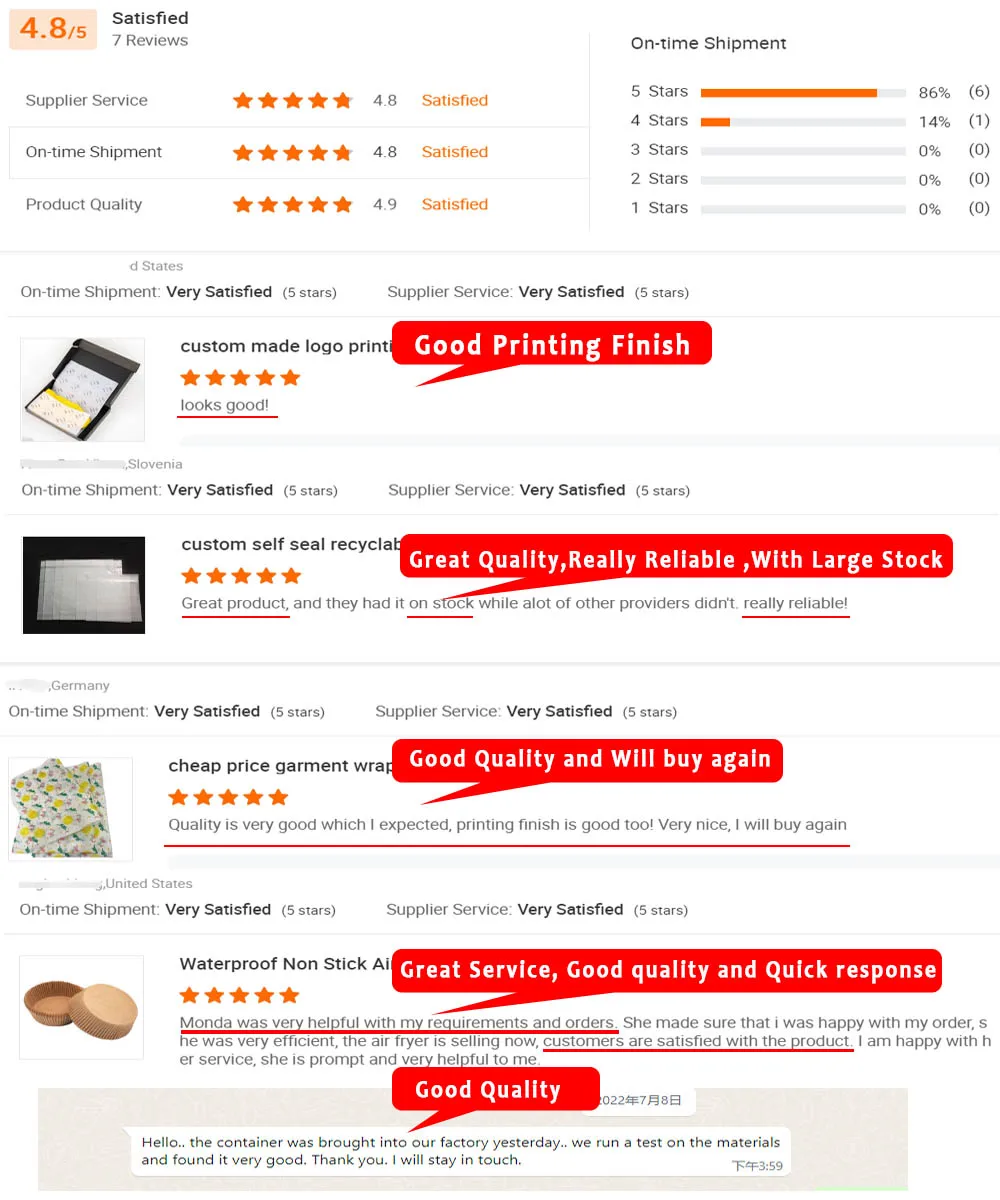The image appears to be a detailed overview from an e-commerce rating site, focused on product and service quality rather than direct purchasing. At the top of the image, prominently displayed in gold or orange-colored text against a lighter orange background, is a rating of 4.8 out of 5. This rating is accompanied by the word "Satisfied" and indicates that there are 700 reviews.

Below this primary rating, several metrics for different aspects of service are shown:
- Supplier Service: 4.8, Satisfied
- On-Time Shipment: 4.8, Satisfied
- Product Quality: 4.9, Satisfied

On the right side, specific rating distributions for On-Time Shipment are illustrated:
- 86% of reviewers gave it 5 stars.
- 14% gave it 4 stars.
- The other rating categories (3 stars, 2 stars, 1 star) have 0%.

Further down, several product listings are featured, each followed by ratings and reviews. Some of the discernible items and their details include:

1. **Custom-Made Logo Printed item (possibly envelopes)**: This product has received 5 stars. Notes mention custom, self-seal, and recyclable attributes, though specific details are hard to discern.
   
2. **Cheap Price Garment Wrap**: This seems similar to wrapping paper and has been rated 5 stars.
   
3. **Waterproof, Non-Stick product**: Specifics are unclear, but it also appears to have a 5-star rating.

Additionally, there are red speech bubble overlays containing customer feedback:
- "Good Printing and Finish"
- "Great Quality, Really Reliable with Large Stock"
- "Good Quality and Will Buy Again"
- "Great Service Quality and Quick Response"
- "Good Quality"

Despite the lack of displayed prices, the ratings and reviews suggest a reliable and highly regarded site, emphasizing quality and satisfaction in service and product offerings.